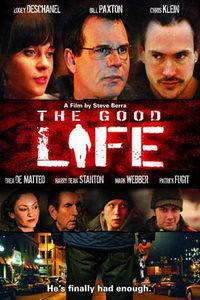The image appears to be a promotional poster for a movie titled "The Good Life." The movie title is prominently displayed in the center in white text with a red hazy outline, with the 'I' in "Life" creatively rendered as a silhouette figure of a man. At the top, there are three main actors featured: a woman on the left, and two men, including Bill Paxton in the center. The other actors at the top include Zooey Deschanel and Chris Klein. Below the title, the poster showcases four additional actors, including two men wearing hats or caps. The credits indicate that the film is by a director named Steve, though the last name is unclear. At the bottom of the poster, there is text over a partial image of a man's lower back and upper thighs, holding a gun, standing in a city street, with the phrase "he's finally had enough" suggesting a pivotal plot point. This detailed composition of images and text suggests it is the front cover of a DVD or movie poster designed to intrigue and attract viewers.